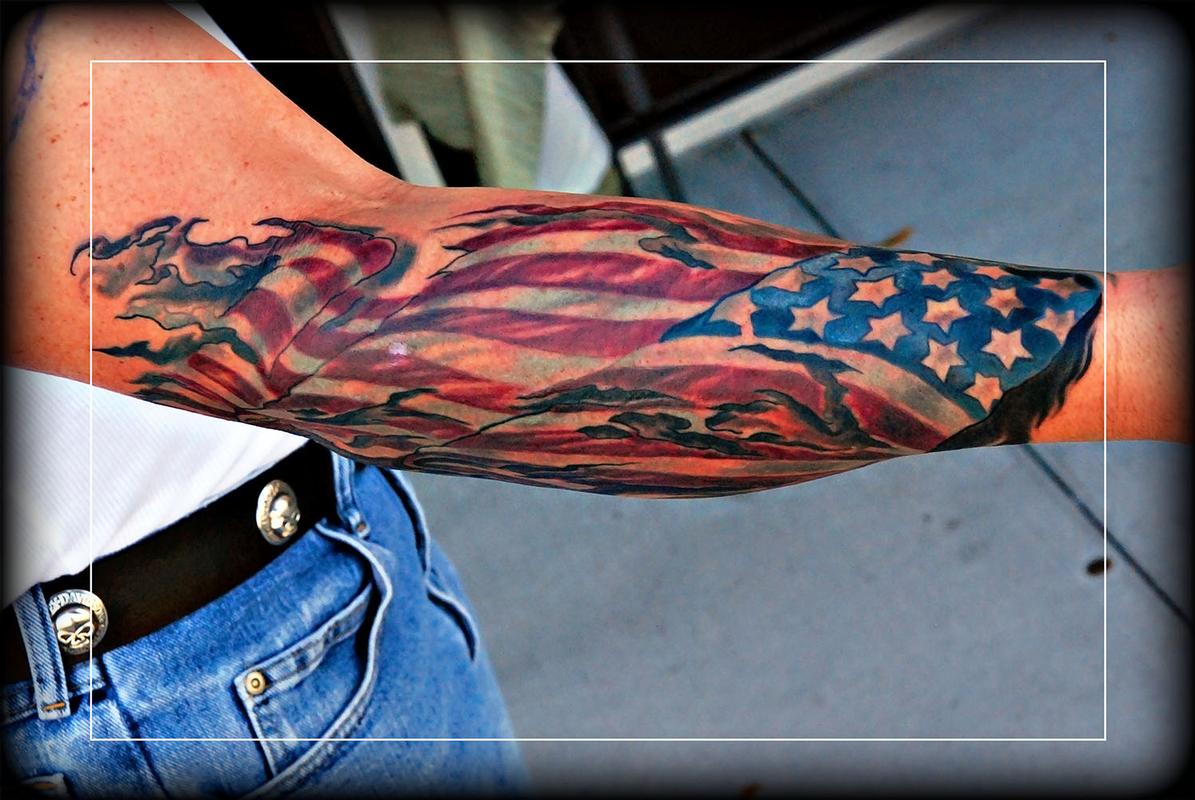In the photograph, a person with fair skin is holding out their right arm, prominently displaying a tattoo of a tattered American flag. The tattoo stretches across the front of the forearm towards the inner arm. The flag features red and white stripes that appear worn and tattered, with black and gray squiggly spots interspersed throughout. The stars are left uncolored, revealing the skin tone underneath, while the blue background of the stars remains intact. The person is dressed in a white top, a black belt adorned with a skull stud, and blue jeans. The background includes a concrete floor and possibly a black or brown wall with white molding, adding to the overall gritty aesthetic. The image itself is framed within a white rectangle outline, creating a clear visual focus on the tattooed arm.